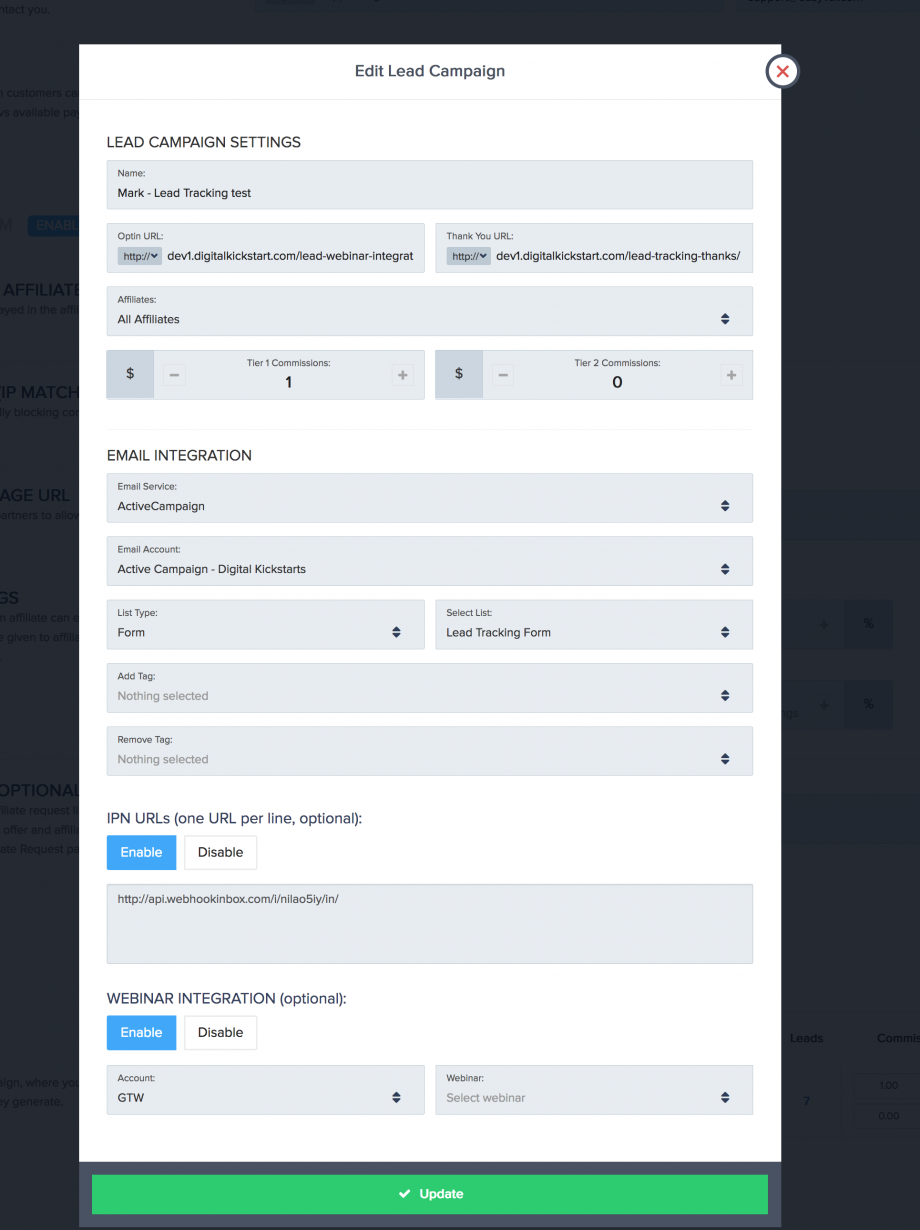A detailed caption for the image described:

"Displayed on a black background, the image shows a computer screenshot of an open white form document, designed for editing a lead campaign. The form is titled 'Edit Lead Campaign' and is structured like a digital piece of paper with various boxes where information can be entered to manage the campaign settings. At the top of the form, under the heading 'Lead Campaign Settings,' there are fields for 'Opt-in URL' on the left and 'Thank You URL' on the right. Below these fields, there is a 'Box for Affiliates' populated with 'All Affiliates.' Further down, two smaller horizontally aligned boxes are labeled 'Tier 1 Commissions' with an entry of '1,' and 'Tier 2 Commissions' with an entry of '0,' both marked with dollar signs to indicate monetary values.

The form continues with five rows intended for additional details: 'Email Integration,' with specified service 'Active Campaign,' followed by 'Email Account' set to 'Active Campaign, Digital Kickstarts.' The 'List Type' is identified as 'Form,' with an adjacent option reading 'Select List Lead Tracking Form.' Additional settings include 'Add Tag' and 'Remove Tag,' both of which are currently unselected.

An area titled 'IP and URLs' allows for one URL per line, displayed as optional. A button labeled 'Enable' in blue with white letters is placed near this section, and a URL 'apiwebhookinbox.com' is filled in. The next section, 'Webinar Integration (optional),' also features a blue button labeled 'Enable.' It includes fields for 'Account' with 'GTW Webinar' and 'Select Webinar.' Finally, the form concludes with a green bar at the bottom, marked 'Update' in white lettering paired with a checkmark, signifying the submission operation."